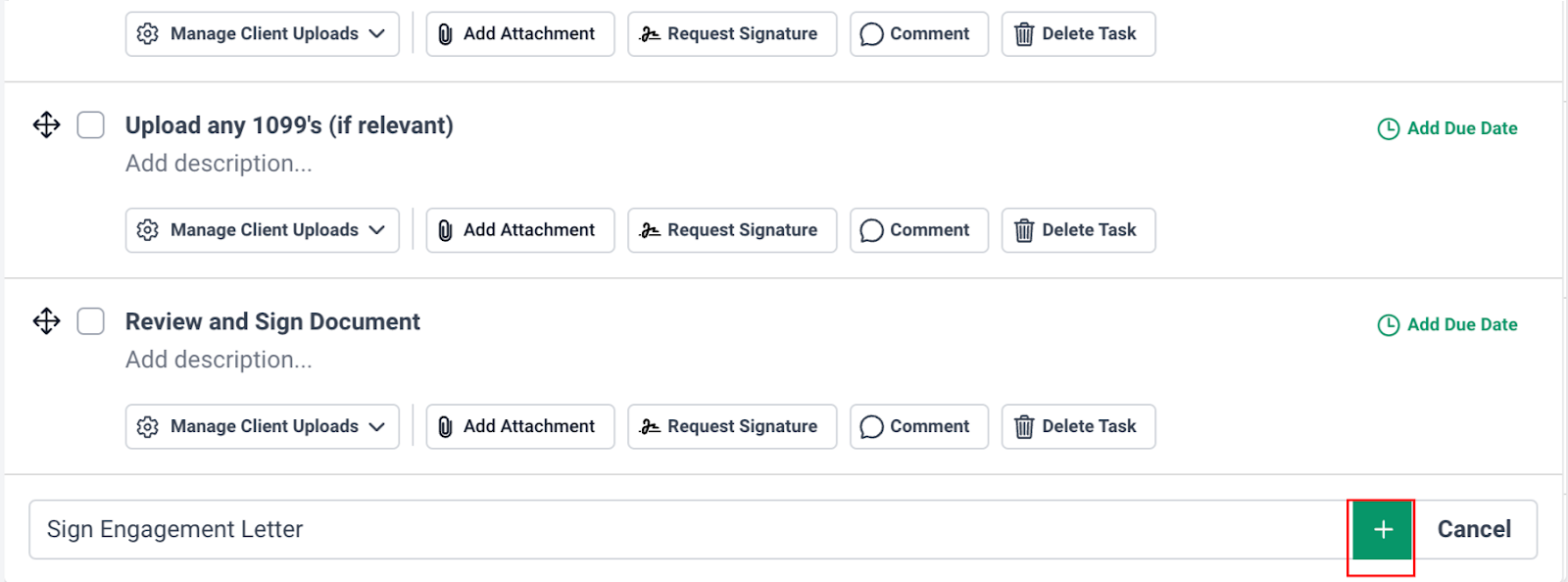This screenshot appears to be from a client management website interface. At the very top, a horizontal series of labeled rectangles is displayed, starting with "Manage Client Uploads" featuring a drop-down arrow. The subsequent options include "Add Attachment," "Request Signature," "Comment," and "Delete Task."

Directly below this menu, there's a gray dividing line. Following the line, an empty rectangular box is labeled "Upload any 1099s" with a note in parentheses that reads "(If Relevant)." Beneath this box is the instruction "Add Description." In the section below, similar options are presented: "Manage Client Uploads" with a drop-down menu, "Add Attachment," "Request Signature," "Comment," and "Delete Task."

Next, there is a section titled "Review and Sign Document," which includes a checkbox on the left and again the instruction "Add Description." Below this, the options "Manage Client Uploads" with a drop-down menu, "Add Attachment," "Request Signature," "Comment," and "Delete Task" reappear.

At the bottom of the interface, the section is labeled "Sign Engagement Letter." To the right of this label, there's a green square featuring a white plus symbol, highlighted with a red box around it to draw attention, likely indicating an actionable button. Further to the right, a white rectangle labeled "Cancel" is present.

Additionally, next to the "Upload any 1099s" and "Review and Sign Document" sections, on their far right-hand side, there is green text that reads "Add Due Date."